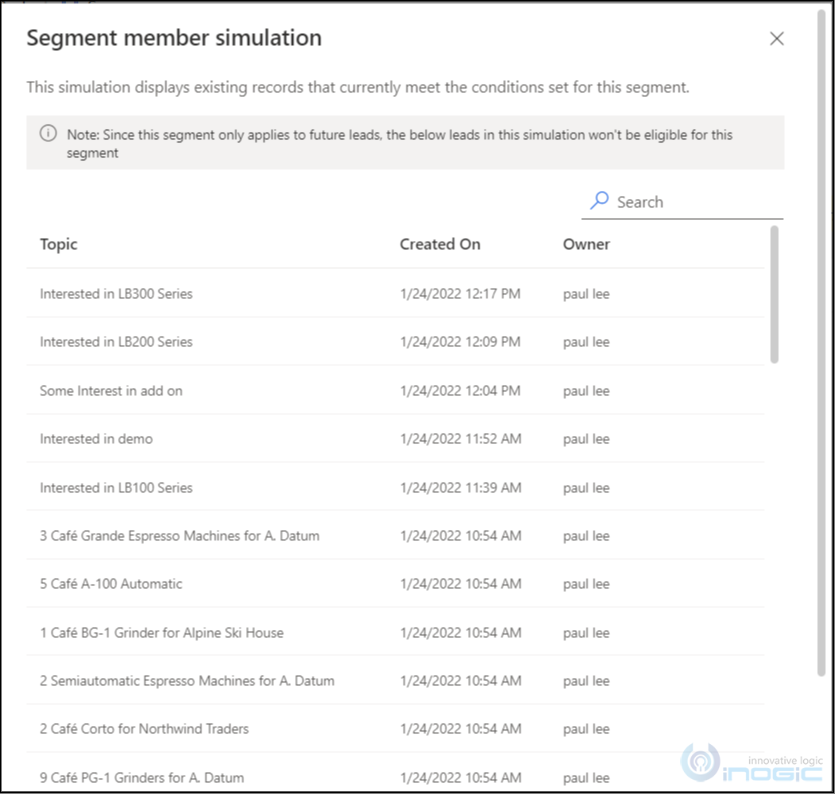This image depicts a website interface with a clean, white background. At the top, bold black text prominently displays the title "Segment Member Simulation" flanked by gray "X" icons on both the left and right sides. Directly below, a gray text message reads: "The simulation displays existing records that currently meet the conditions set for the segment." 

A light gray box follows, containing darker gray text that states: "Note: Since this segment only applies to future leads, the below leads in this simulation won't be eligible for this segment." 

Continuing downward, a list section is present. Above this list is a small search bar featuring a blue magnifying glass icon. The list headers, spelled out in black letters, include "Topic," "Created On," and "Owner." The list entries provide specific details such as:
- "Interested in LB 300 series on 1-24-2022 at 12:14 p.m.," with ownership attributed to Paul Lee.
- Various similar entries follow, culminating with the last entry: "9 Cafe PG-1 Grinders for adatum on 1-24-2022 at 10:54 a.m.," also from Paul Lee.

Entries appear in reverse chronological order, with the most recent at the top. In the bottom right-hand corner, there's a watermark resembling a logo in a blue hue stating, "Innovative Logic In Object."